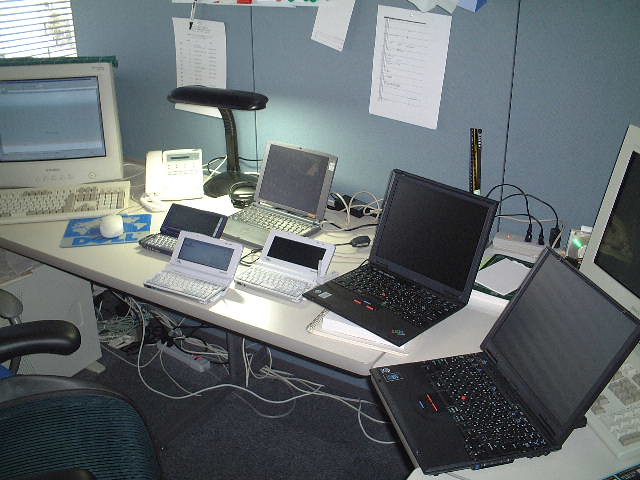The image depicts a well-equipped office space with a white desk against grayish light blue walls. There is a combination of six laptops and two desktop computers. The laptops vary in size and color: three are large with two in black and one in silver, and three are miniature with one each in black, white, and silver. To the left of the desk, a rotary phone, a computer monitor with an attached wired keyboard, and a black desk lamp are visible. The desk also holds a mouse pad with a blue and gray design, and a wired mouse. Above the desk, pieces of paper are affixed to the wall, and a window with blinds pulled up lets in natural light. The floor is covered with dark carpeting and features an electrical power supply with numerous cords beneath the desk. There are both a lighter blue chair in front of the desk and a darker chair off to the side. The desk exudes a sense of organized chaos typical of a busy workspace.